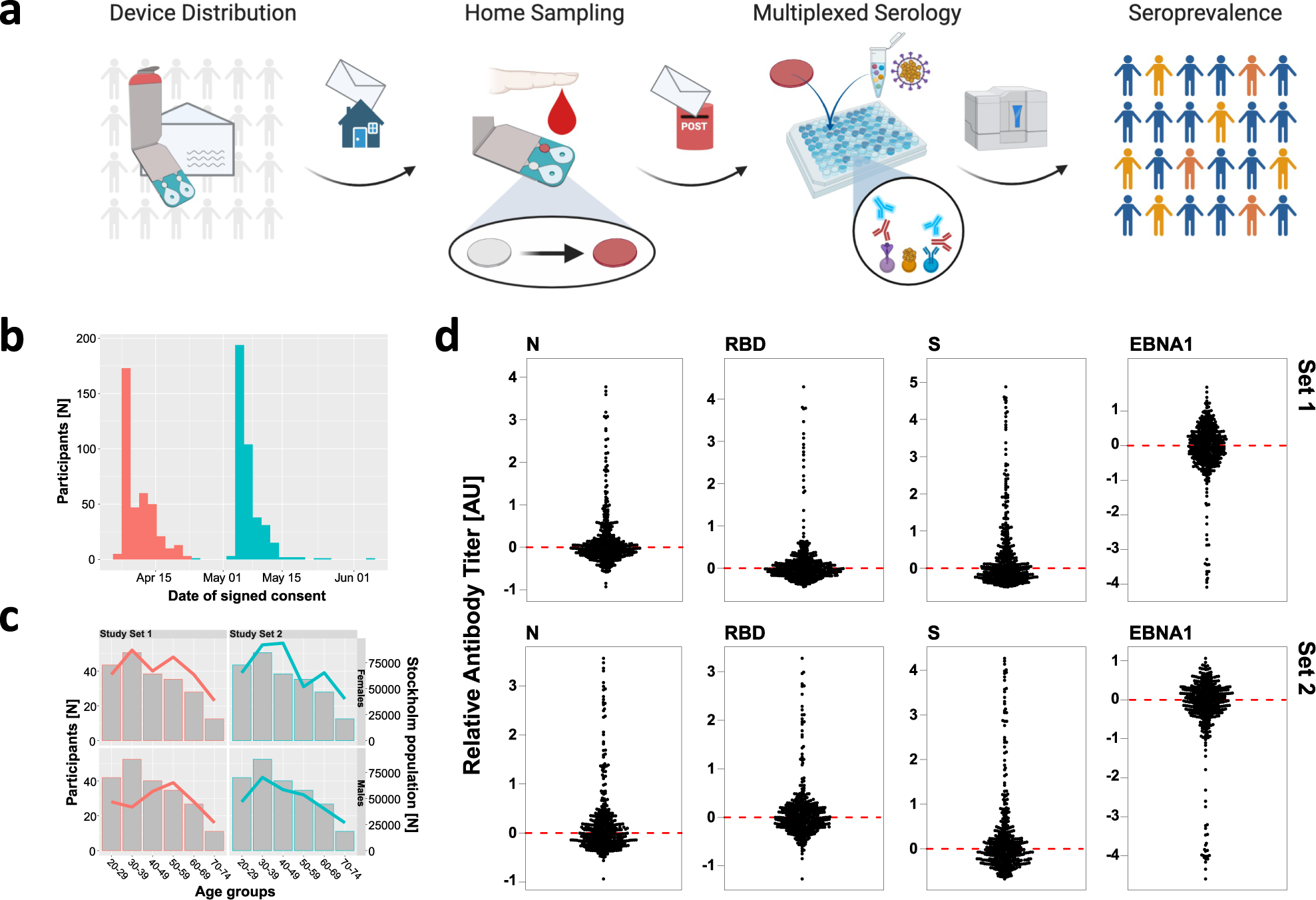The image is a detailed infographic illustrating a step-by-step procedure for a scientific study involving device distribution, home sampling, and serological testing. At the top, section A features labeled subsections: "Device Distribution," showing an envelope with a group of stick figures holding hands, symbolizing participants receiving devices via mail. The next stage depicts "Home Sampling," with an arrow leading to an envelope next to a house, indicating the collection of blood samples at home. Following this, "Multiplexed Serology" and "Seroprevalence" are represented with further diagrams and charts showing blood collection and testing processes.

Section B is a bar chart highlighting participant data, with the y-axis labeled "Participants" and the x-axis labeled "Date of Signed Consent." 

Section C presents another bar chart with "Participants" on the y-axis and "Age Groups" on the x-axis, showing a declining trend with increasing age groups. 

Section D, located at the bottom, comprises multiple detailed readouts labeled "Relative Antibody Titer (AU)," featuring two sets of results ("Set 1" and "Set 2") and additional indicator markers such as "N," "RBD," "S," and "EBNA1." The accompanying graphs and lines illustrate various serological data trends. The entire layout includes red, blue, and gray colorations for the graphs and diagrams, enhancing the visual differentiation of data points and trends.